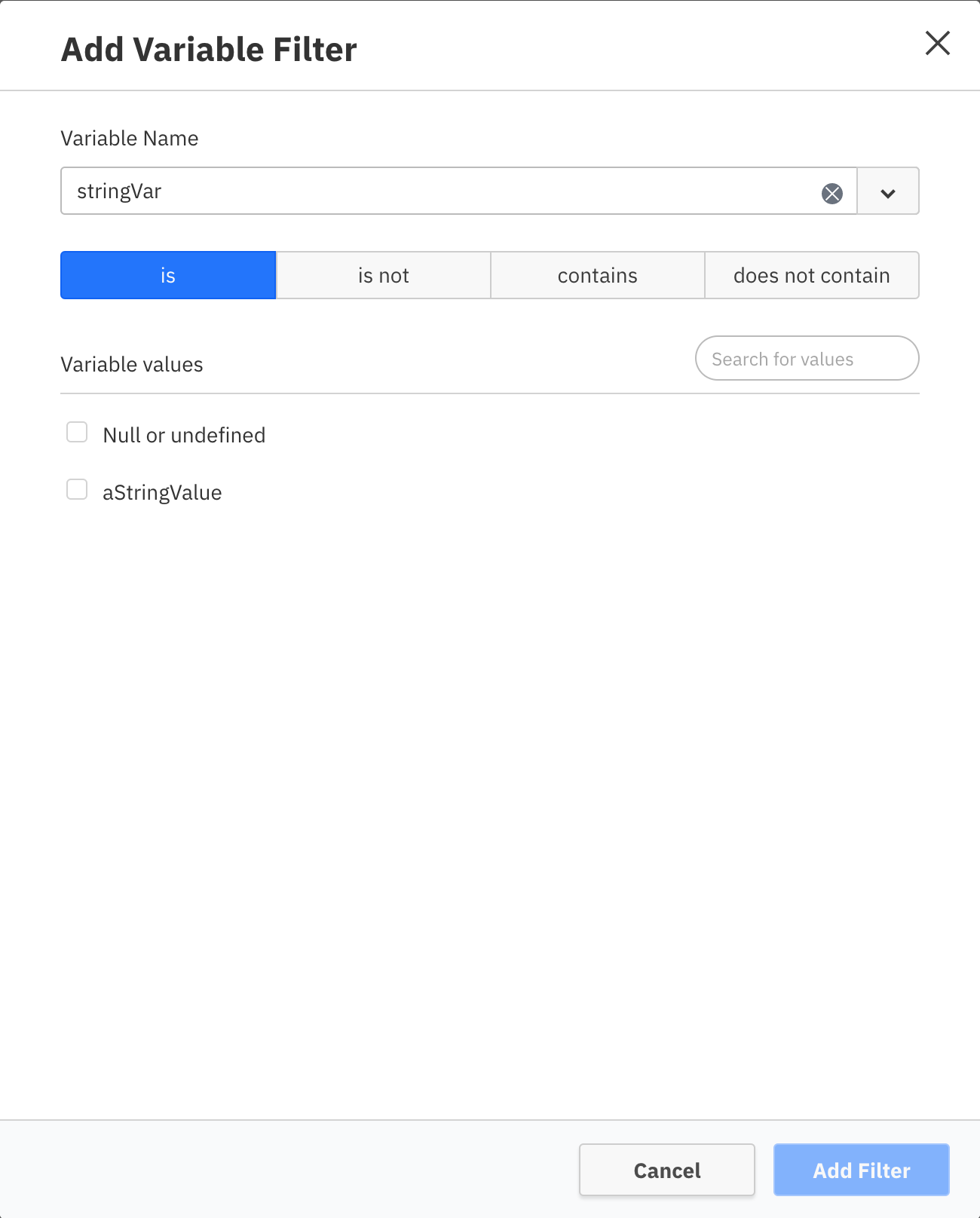The vertically rectangular image features a clean, all-white background. At the top, a thin black horizontal line divides the header from the body of the window. Directly beneath this line, aligned to the left, is bold and enlarged text reading "Add Variable Filter". On the right-hand side of this header, there is an "X" icon for closing the window.

Following this is another thin, light grey horizontal line, creating a distinction between the header and the main content. Underneath, left-aligned, is the label "Variable Name," followed by a drop-down menu for selecting a variable. Below this menu, three side-by-side filter options are displayed: "is," "is not," "contains," and "does not contain." The "is" option is currently selected, highlighted in blue.

Further down, a section labeled "Variable Values" appears, alongside a search box for finding specific values. This section is also separated by a thin grey horizontal line. Beneath it, there are two selectable items: "null or undefined" and a string value, both displayed with checkboxes.